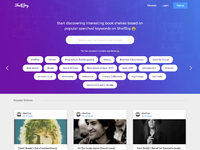The image displays a blurred and low-resolution screenshot of a website with a predominantly purple and white color scheme. The upper half features a gradient background blending purple and blue hues. A prominent white search box is centrally located, suggesting users can input queries. In the top right corner sits a blue button, though the text is indiscernible. Surrounding the search box, a multitude of white circular icons likely represent various categories, with approximately twenty visible. Arrows flanking this section imply additional categories can be accessed by navigation.

Transitioning to the bottom half, the background shifts to gray, showcasing three individual Instagram-style posts. The first image depicts a person with short, curly hair and light-colored hair, their gender ambiguous due to the blurry resolution. The second image presents a man with a broad smile and black hair. The third image features a woman wearing a hat, long hair flowing, holding her hands close to her chest. The identities of these individuals remain unclear, as do the specific purposes and offerings of the website due to the overall image clarity.